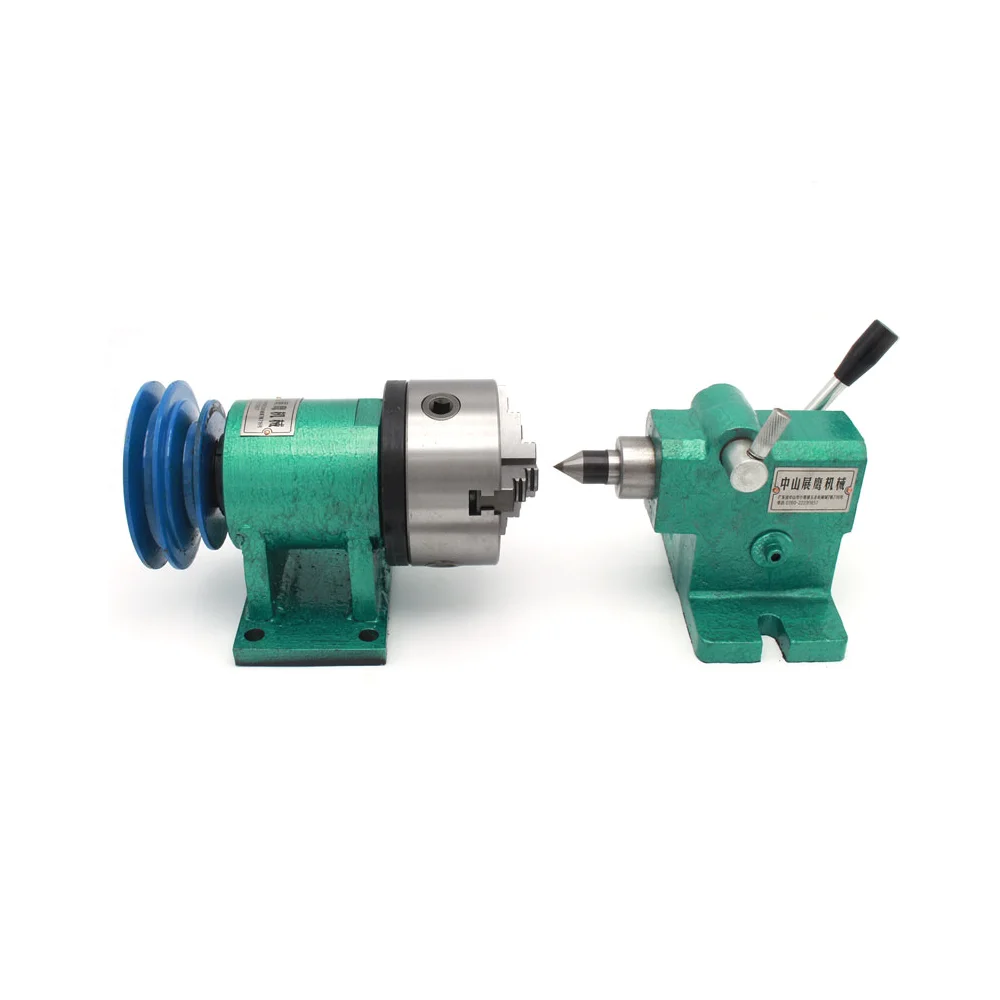This photograph showcases two pieces of intricate factory equipment positioned against a stark white background. The apparatuses are predominantly burnished aqua blue with gray shadowing. The larger machine sits on the left, featuring a green cylindrical metal piece mounted on a matching flat base. Attached to this cylinder are three royal blue rings, which protrude from the left side. Extending to the right of the green cylinder is a stainless steel cylinder, separated by a black segment with a hole at the top. The machine also includes a silver-toned metal label and two holes likely for mounting onto a workbench.

The right-side equipment, also a green hue, consists of a rectangular base of the same color. A stainless steel circular piece emerges from the left side of this base, transitioning into a pointed element akin to a solid steel pen tip, encircled by a black component. Directly behind this pointed section is a black lever connected to a steel shaft. The equipment is marked with Asian writing on a label, indicating its origin or purpose. The combination of manual handles, steel components, and intricate design elements suggests these machines are crafted for precise industrial tasks.